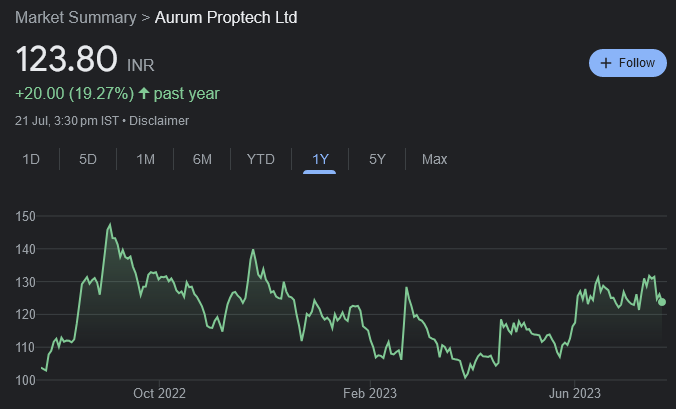This is a mobile screenshot displaying a financial graph in dark mode, with a charcoal black background. In the top left corner, the text "Market Summary" appears in gray font, followed by a forward arrow. Next to it, in white font, is the label "AURUM PropTech LTD." To the right, there is a blue oval with a black plus sign and the word "Follow," indicating an option to follow the stock. 

Beneath this, the stock value is stated as "123.80 INR," with a growth of +20%, reflecting a 19.27% increase over the past year. The date "21 July 3:30 p.m. IST" and a "Disclaimer" follow this information. A menu below these details offers various time frames for the graph: "1D" (one day), "5D" (five days), "1M" (one minute), "6M" (six months), "YTD" (year to date), "1Y" (one year), "5Y" (five years), and "MAX" (maximum). The selected time frame is "1 Year."

The graph itself, positioned below the menu, displays values on the vertical axis ranging from 100 to 150, with 100 at the bottom and 150 at the top. Along the horizontal axis, the dates are marked: October 2022, February 2023, and June 2023.